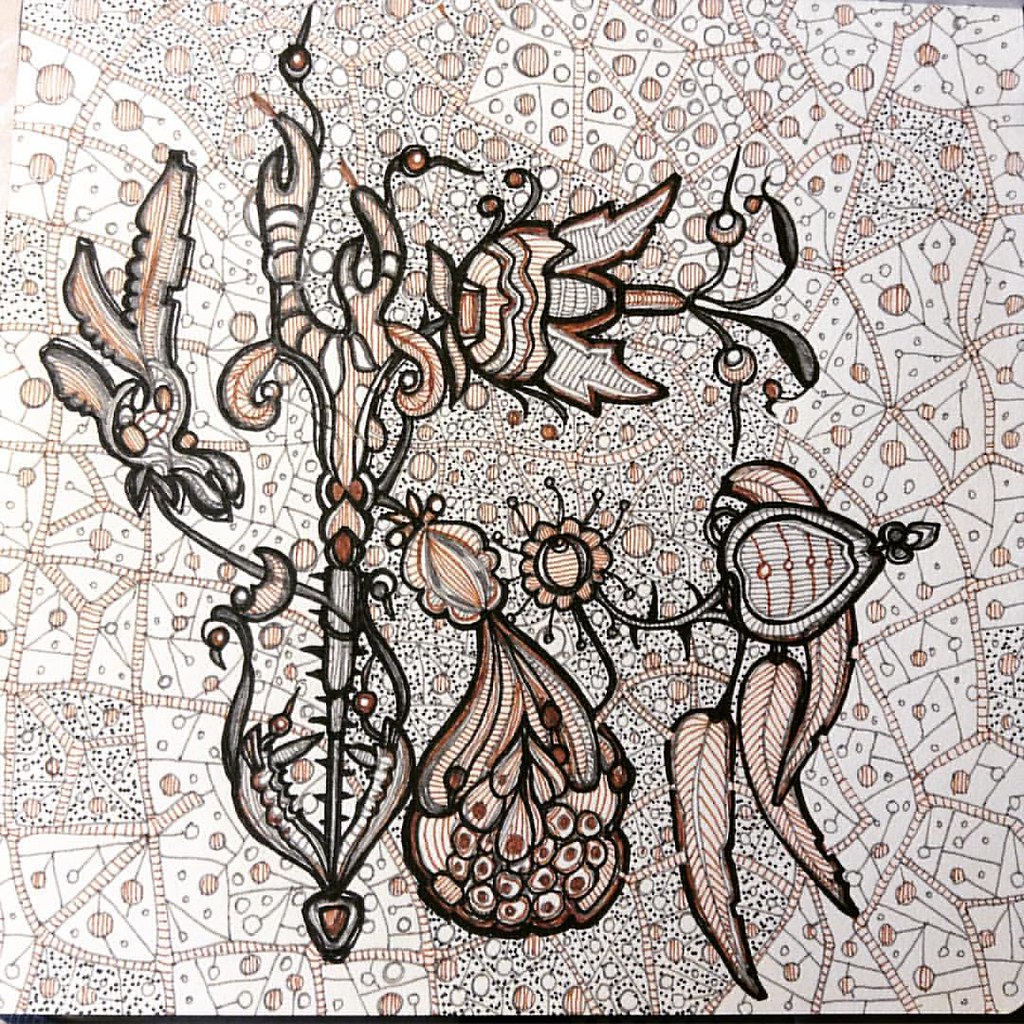This image is a highly intricate artwork with a complex, almost cellular pattern reminiscent of a microscopic view of cells. The background features a mix of black, white, beige, and dark brown hues, providing a richly detailed canvas. Throughout the image, there is a repeating motif of interconnected sections that resemble squares or various polygons, each containing intricate lines and circular designs.

Prominent within these sections are large circles adorned with red or orange stripes, and smaller white circles, all interconnected by black lines that also link them to the section borders. These borders are thick, slashed through horizontally, creating an additional layer of patterning. 

In the center of the artwork lies an alien-like floral design, with leaves and buds that appear both intricate and menacing, reminiscent of eyes or sharp claws, and resembling carnivorous plants. These elements, composed primarily of dark, earthy tones like browns and reds, add an eerie, dynamic quality to the piece.

Scattered throughout are black polka dots and small black circles, some with orange lines, contributing to the overall complexity. Larger shapes that look like feathers or pears in brown and beige hues further enhance this artwork's intricate and mesmerizing detail.